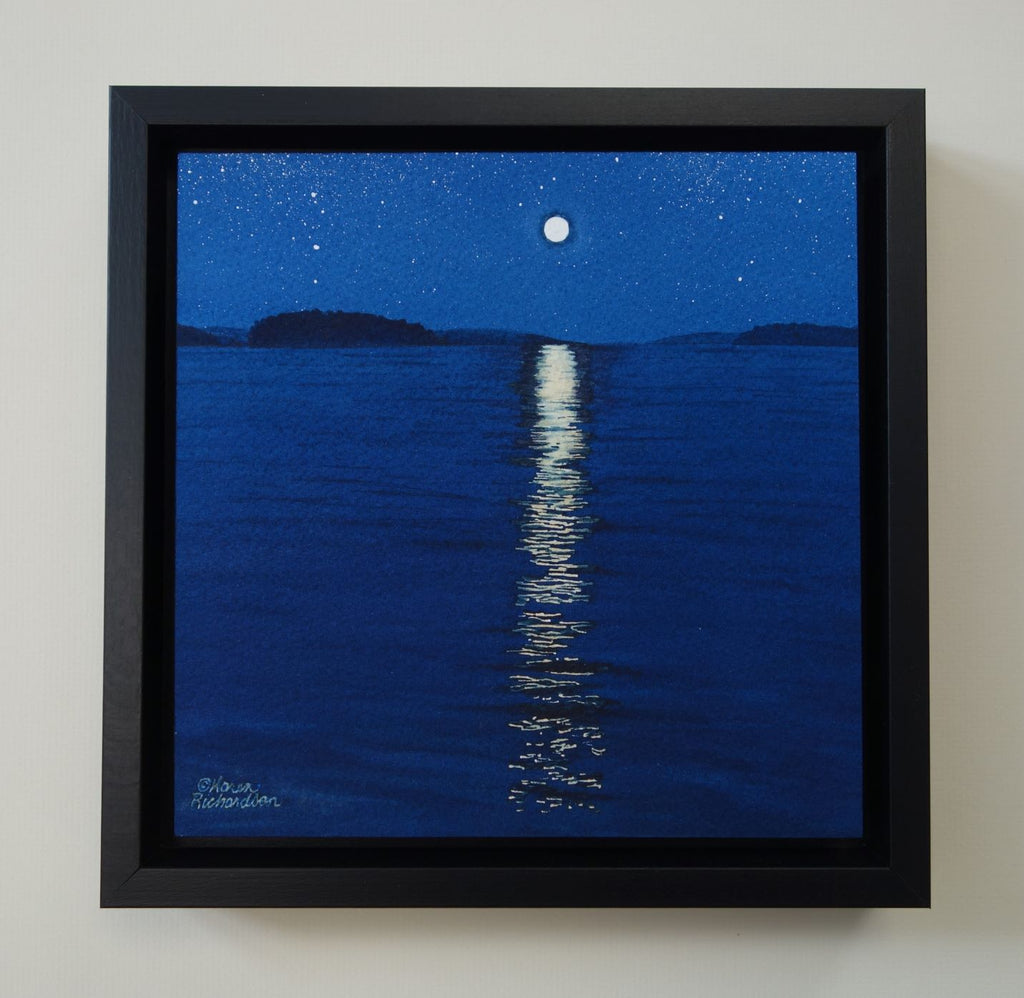This image, which resembles a painting, is framed in a simple, thick black frame and hangs on a plain white wall, casting a shadow to the right. The painting is square and captures a serene nocturnal scene. The deep blue water, which makes up most of the lower portion, exhibits subtle ripples and waves. Above the water, a slightly off-center full moon glows white with a subtle amber hue, its light reflecting in a shimmering line down the center of the water. The moonlit night sky is filled with stars, transitioning from a deep to lighter blue, and framed by a distant horizon that's dotted with the silhouettes of hills or trees. The painting features a black border before the main image, and small, hard-to-read text in the bottom left corner.